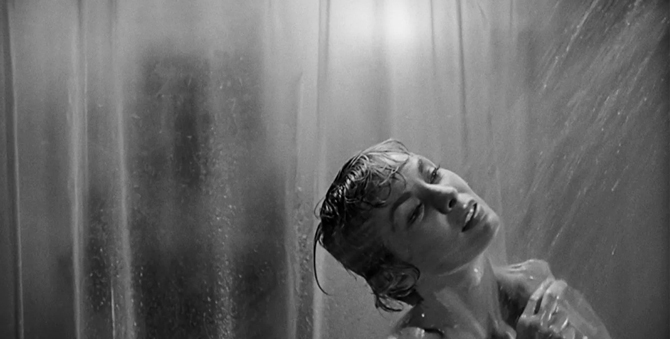This black-and-white image captures the iconic shower scene from the movie "Psycho." The photograph, presented in a horizontal format with a ratio of approximately 1 to 2.35, likely indicates it’s a movie still. The central focus is a female character in mid-shower, with droplets cascading down her face, wetting her hair, face, shoulders, and neck. Despite a slight blur, hinting at it being a screenshot, the details are vivid: water flows from the top right of the image, while a concentrated highlight illuminates the top center, casting a dramatic light on the woman. Her expression suggests she is deep in thought, adding a psychological depth to the scene. The background is dominated by a shower curtain with a notable shadow of a person standing behind it, obscured by a misty fog, enhancing the sense of suspense. The light and shadows interplay, leaving the woman's right side in darkness and her left side lit, drawing viewers into the chilling and tense atmosphere of this legendary film moment.